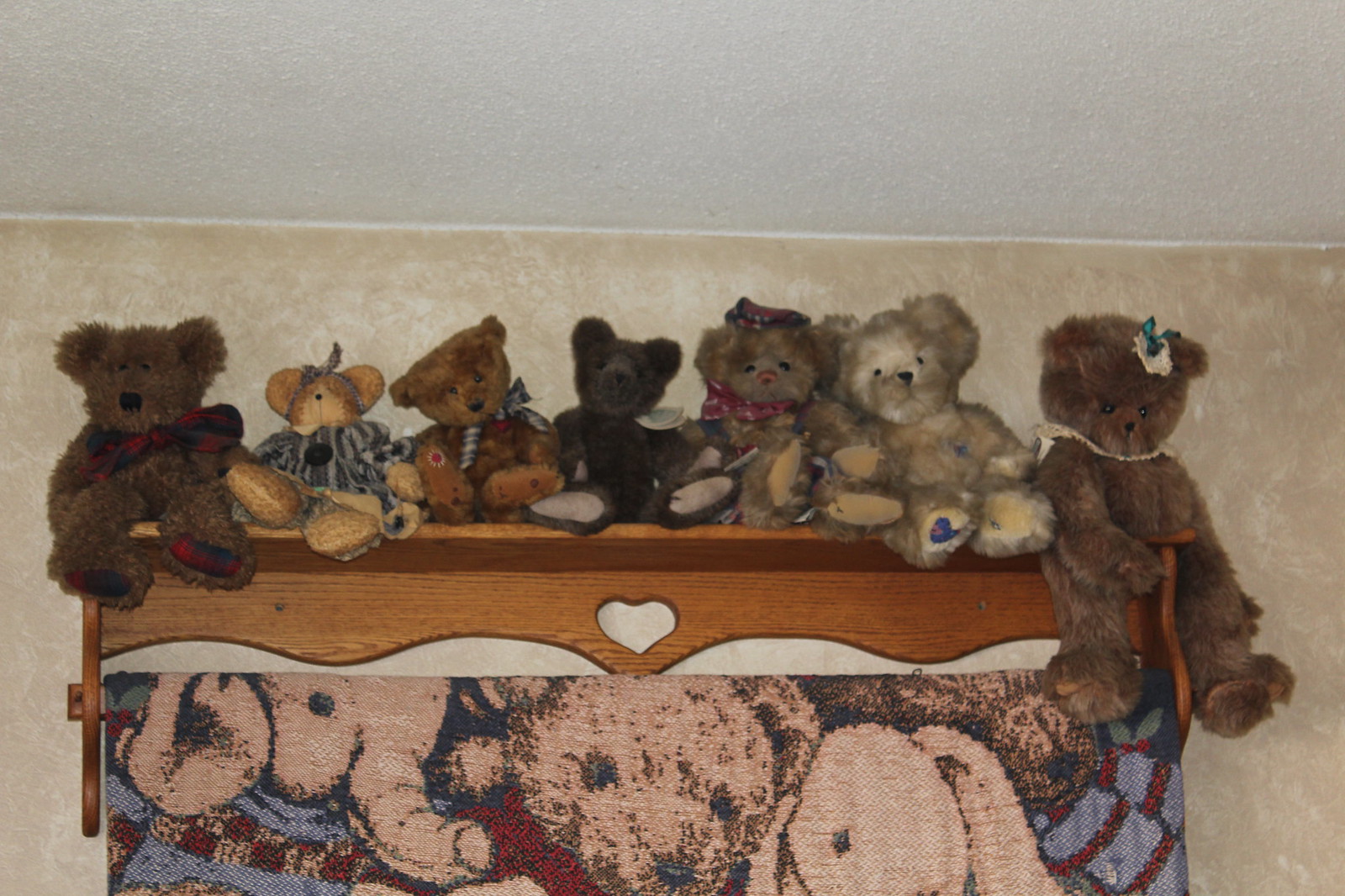This photograph captures a cozy, whimsical scene featuring seven distinct teddy bears perched atop a wooden shelf, also functioning as a towel hanger. The shelf, adorned with a heart-shaped cutout, reveals the beige-tan wall behind it, ornamented with white splotches creating a subtle pattern. The shelf is mounted high on the wall, with the teddy bears' heads sitting just about half a ruler's length below the white, popcorn-textured ceiling. Each teddy bear differs in color and size, ranging from various shades of brown and tan to some with bows while others do not. Below the shelf, a woven throw blanket featuring an elephant, a bear, and a bunny head in a palette of red, beige, light brown, and blue can be partially seen, further enhancing the playful ambiance of the setting.